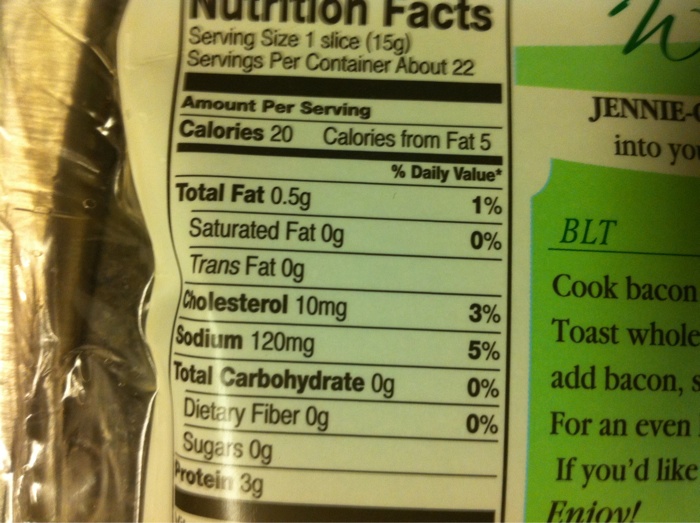This is a detailed close-up photograph of a package of food, specifically bacon or potentially imitation bacon, although the exact type is unclear. The image prominently displays the nutrition facts against a yellowish background with black font. Each serving size is listed as one slice (15 grams), with approximately 22 servings per container. Nutritional details per serving are as follows: 

- Calories: 20
- Calories from fat: 5
- Total fat: 0.5 grams
- Saturated fat: 0 grams
- Trans fat: 0 grams
- Cholesterol: 10 milligrams
- Sodium: 120 milligrams
- Total carbohydrate: 0 grams
- Dietary fiber: 0 grams
- Sugar: 0 grams
- Protein: 3 grams

To the right of the nutritional information, there is a partially visible section that includes usage instructions and a recipe suggestion to make a BLT. The instructions mention cooking the bacon or toasting, and implied additional steps to complete the preparation, although some text is cut off and not fully readable. The brand name "Jenny O" is partially visible, indicated as the producer of this bacon product.